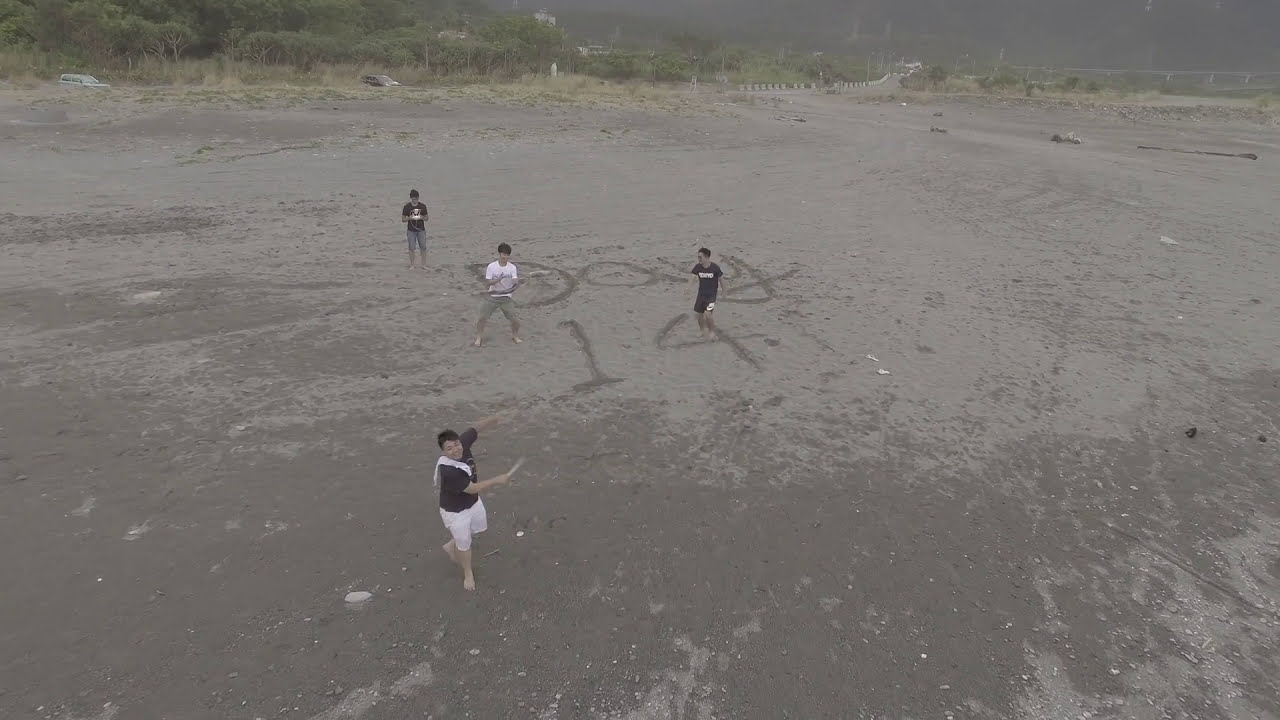The image captures an outdoor scene on a beach area with a distinct dull and grayish-brown sandy terrain that stretches into the distance, where lush green trees subtly emerge through a slight, gray fog. In the foreground, four individuals—three men and one woman—are engaged in animated activities. The woman, identifiable by her white sash, black t-shirt, and white shorts, appears to be turning swiftly, possibly to catch something. The three men around her are attired in varied combinations of black and white shirts with blue or black shorts, one brandishing a stick as if waving it towards the camera. All of them have their attention captured by a drone overhead, which is likely responsible for taking the photo. Central to the sandy expanse, the words "Day 14" are inscribed, evidencing their interaction with the environment. Flanking the scene, two parked cars and a dirt road with pillars add to the ambiance of a leisurely, slightly overcast day marked by casual play and subdued tones.